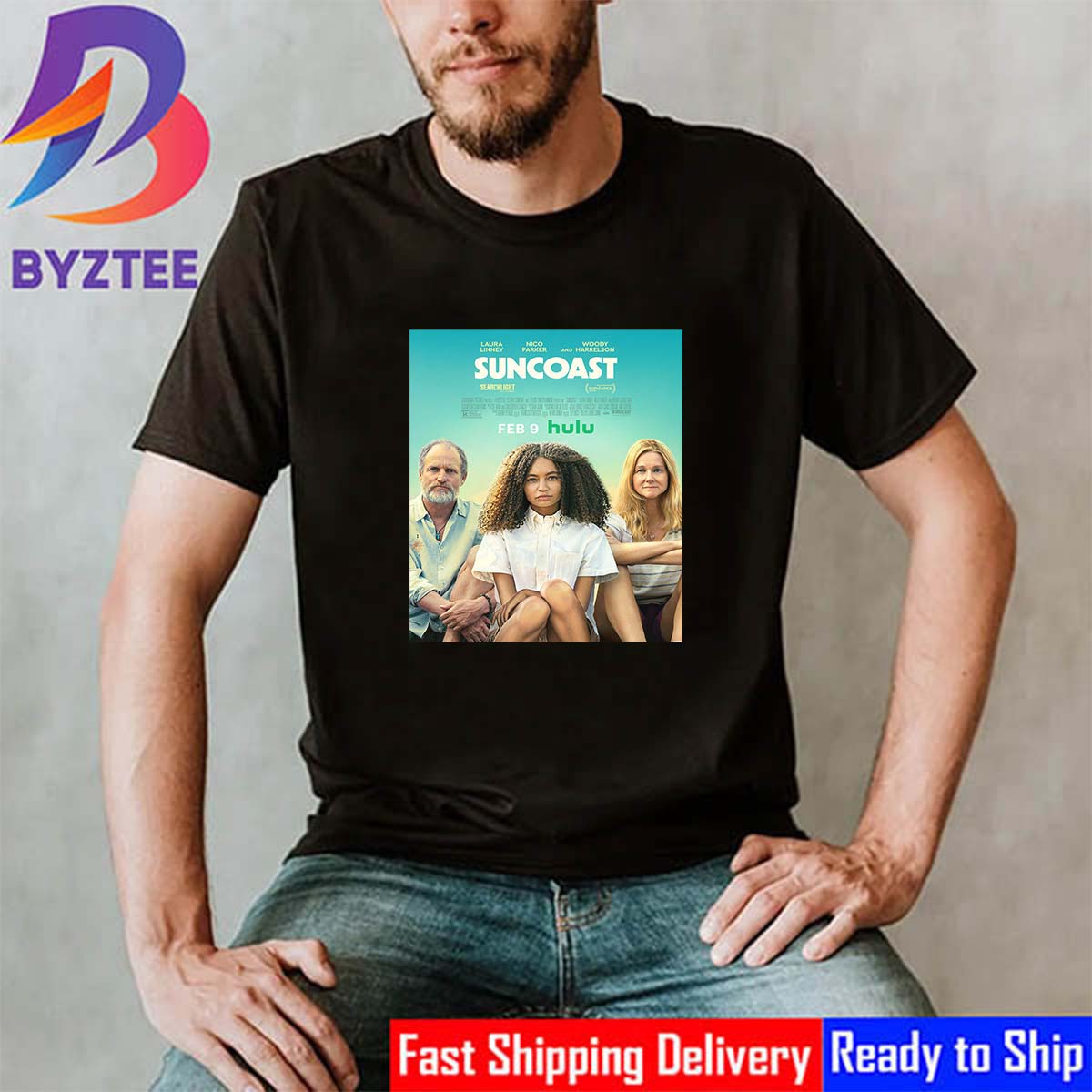This image features a man partially obscured, showcasing a visible bearded part of his face. He is dressed in a black t-shirt paired with blue jeans, sitting with his hands resting just below his waist. Prominently displayed on his t-shirt is a blue square graphic, which at the top reads "Suncoast" in white letters, and below that, "Hulu." The graphic includes an image of three people seated, promoting the Hulu show "Suncoast," starring Laura Linney, Nico Parker, and Woody Harrelson. The t-shirt also mentions the show's premiere date, February 9th, and depicts a girl with thick, shoulder-length curly hair sitting between Harrelson and Linney.

In the image's upper left-hand corner, there is a swirl of red, blue, and orange colors descending from the top left towards the left center. Beneath this swirl are the letters "B-Y-Z-T-E-E" in purple, above a logo shaped like a 'B' with the top half in purple and the bottom half transitioning from pink to orange. In the bottom right corner, a banner with alternating red and blue backgrounds reads, “Fast Shipping Delivery, Ready to Ship.”